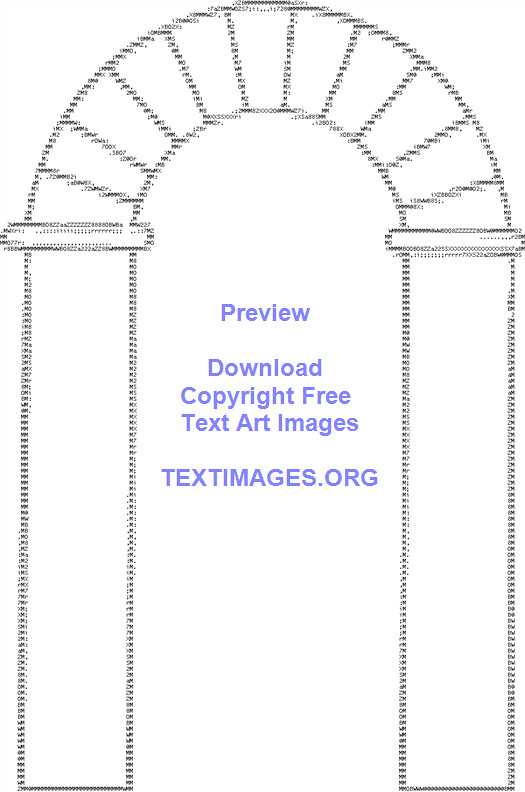The image features a pixelated, outlined arch with a white background. The arch is composed of small, distinct characters like "zeros", "eights", "twos", and "lowercase a's," giving it a rough, "fuzzy" appearance up close but forming a coherent structure from a distance. The sides of the arch consist of vertical rectangular columns, while the top is made of wedge-shaped segments, resembling interlocking stones. Vertical lines, approximately ten in total, span the arch from the left side to the right. 

In the center of the arch is blue text that reads "Preview," "Download," "Copyright Free," and "Text Art Images." Beneath this centered main text, in all caps and also in blue, the website "TEXTIMAGES.ORG" is displayed. This text is clear and not pixelated, contrasting with the pixelated arch graphic.